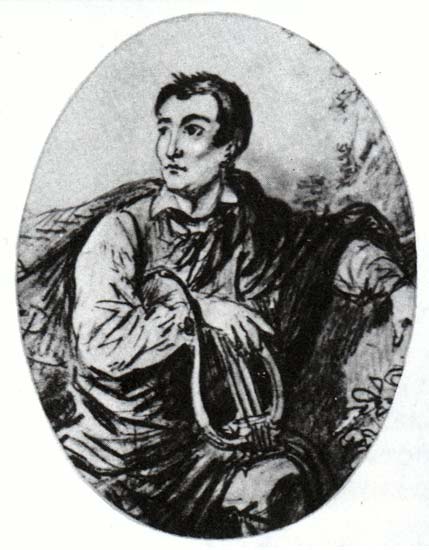This is an oval-shaped black and white sketch, possibly drawn with pencil or ink. It features a man seated in the center, facing the viewer while looking off to his right. His short, slightly spiky brown hair and thick bushy eyebrows stand out against the grayish white background. The man is dressed in a long-sleeve top, from which a collar protrudes at his neck, and he appears to be wearing pants. Draped over his shoulders is a cape or cloak. His left arm rests on an unseen surface, possibly a chair or sofa, while his right arm, bent at the elbow, holds a small musical instrument—a lyre or harp with a horseshoe shape and a few visible strings—which rests on his left thigh. Only the top of his bent right knee is visible in the portrait, and some twigs can be seen in the upper right section of the background. A signature, which may read "Zoe," appears to be located near his right arm.